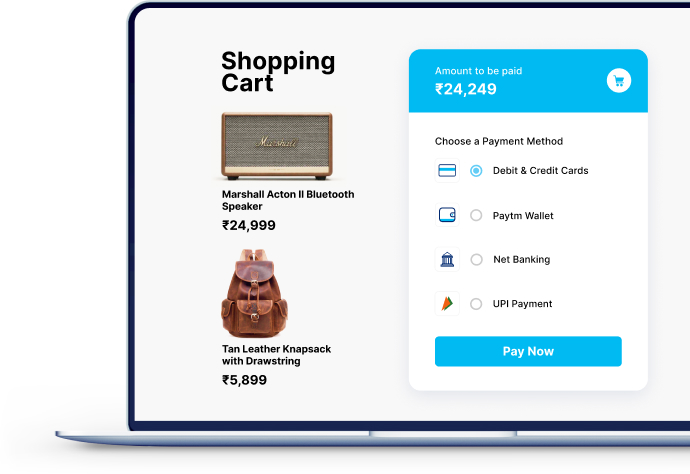The image depicts a detailed online shopping cart listing. At the top, there's a Marshall Action 2 Bluetooth speaker priced at $24,999. The speaker features "Marshall" prominently emblazoned in gold letters across its center. Directly below the speaker listing is a tan leather knapsack with a drawstring, priced at $5,899. 

To the right, the payment section is visible. It starts with a blue banner indicating the total amount to be paid: $24,249. Below this banner, the instructions "choose payment method" are written. A series of icons and buttons for various payment options follow: the first option is for debit and credit cards, then Paytm Wallet, followed by net banking, and finally UPI payment. The section concludes with a smaller blue banner at the bottom featuring the text "pay now" in white lettering.